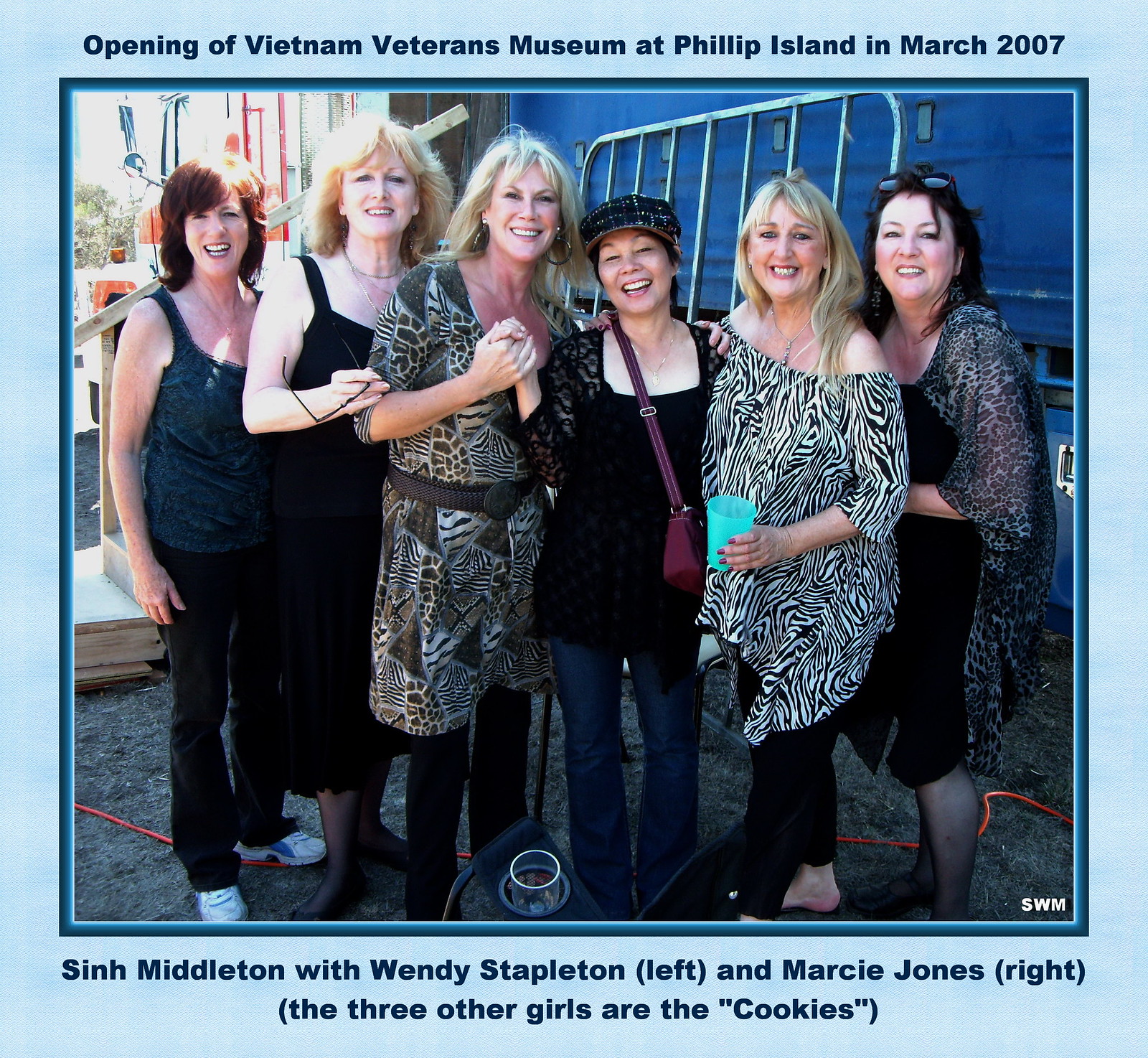The image captures a lively scene of six women in their 40s and 50s, standing shoulder to shoulder and smiling warmly at the camera. They are positioned in front of a truck with a blue trailer, suggesting they are outdoors, possibly at a festival or an event. The text on the image reads "Opening of Vietnam Veterans Museum at Phillip Island in March 2007," and lists the names of the women beneath, identified from left to right.

Starting from the left, the first woman, Sin Middleton, has auburn brown hair, a green tank top, dark-colored pants, and white tennis shoes. Next to her, Wendy Stapleton sports blonde hair and a black dress that falls below the knee, featuring tank top-style straps. To her right is Marcy Jones, who also has blonde hair and is wearing a gray top adorned with various animal print patterns arranged in triangles (cheetah, zebra, and tiger), paired with black pants. 

The middle woman, who appears to be of Asian descent, is smiling and wearing a distinct hat along with a visible purse. To her right, another woman dons a zebra-print dress with black pants. The woman on the far right is wrapped in a leopard-print shawl over a black dress. All six women exude joy and camaraderie, vividly captured in this daylight photo taken at a significant event dedicated to honoring Vietnam veterans.